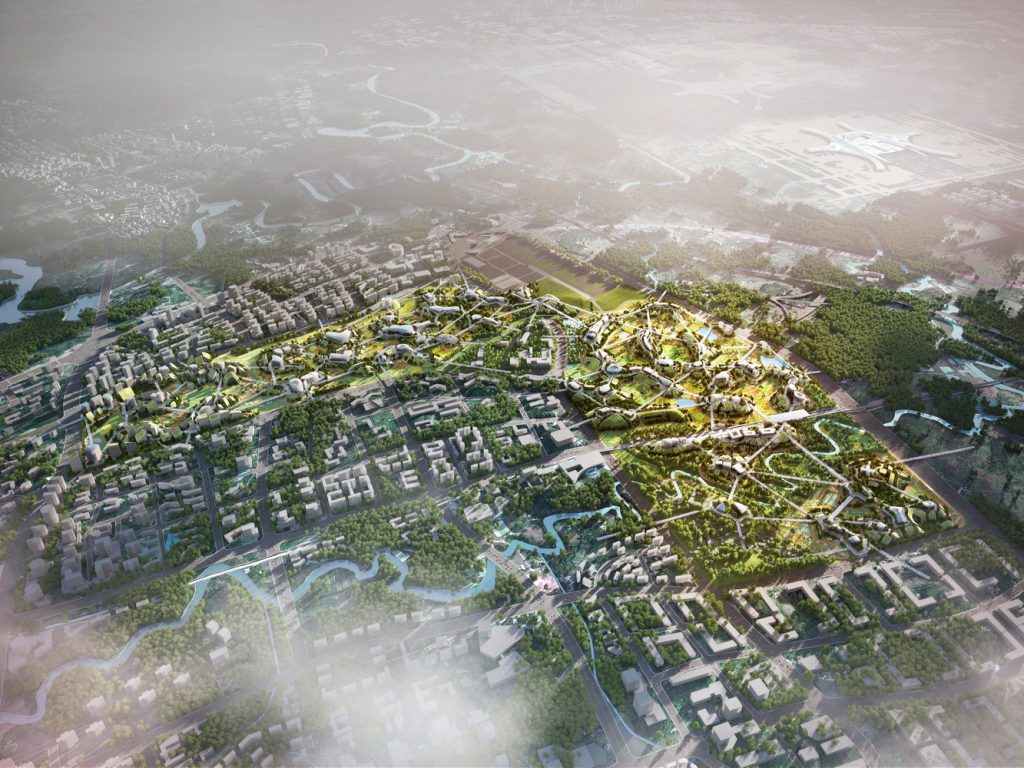This image appears to be an aerial or satellite view of a landscape, possibly computer-generated due to the vivid coloration and intricate design that suggests the influence of AI. The scene includes an expansive area of land with various elements visible from a high vantage point. In the foreground and background, there are hazy clouds that bracket a clearer central section of the image.

The landscape below is dominated by a network of zigzagging roads that crisscross the entire area, connecting various buildings. Many of these structures are peculiar in appearance, likely made of cement and possibly industrial or agricultural in nature, although there are suggestions of residential areas on the left. However, the exact nature of these buildings is difficult to discern due to the altitude of the image.

There are two prominent rivers flowing through the scene, characterized by strikingly blue water that contributes to the artificial feel of the image. One river courses from the bottom left, meanders upwards and towards the center before disappearing into the haze. The second river starts at the top center left, snakes its way to the right and upwards, eventually being obscured by the clouds.

The green landscape is peppered with trees and patches of grass, adding a natural element to the predominantly built environment. On the top right, partially visible through the clouds, there is a large structure that could be an airport or similar complex.

Overall, the image presents a detailed overhead view of a diverse and sprawling landscape, blending natural and man-made elements under a partially cloudy sky.